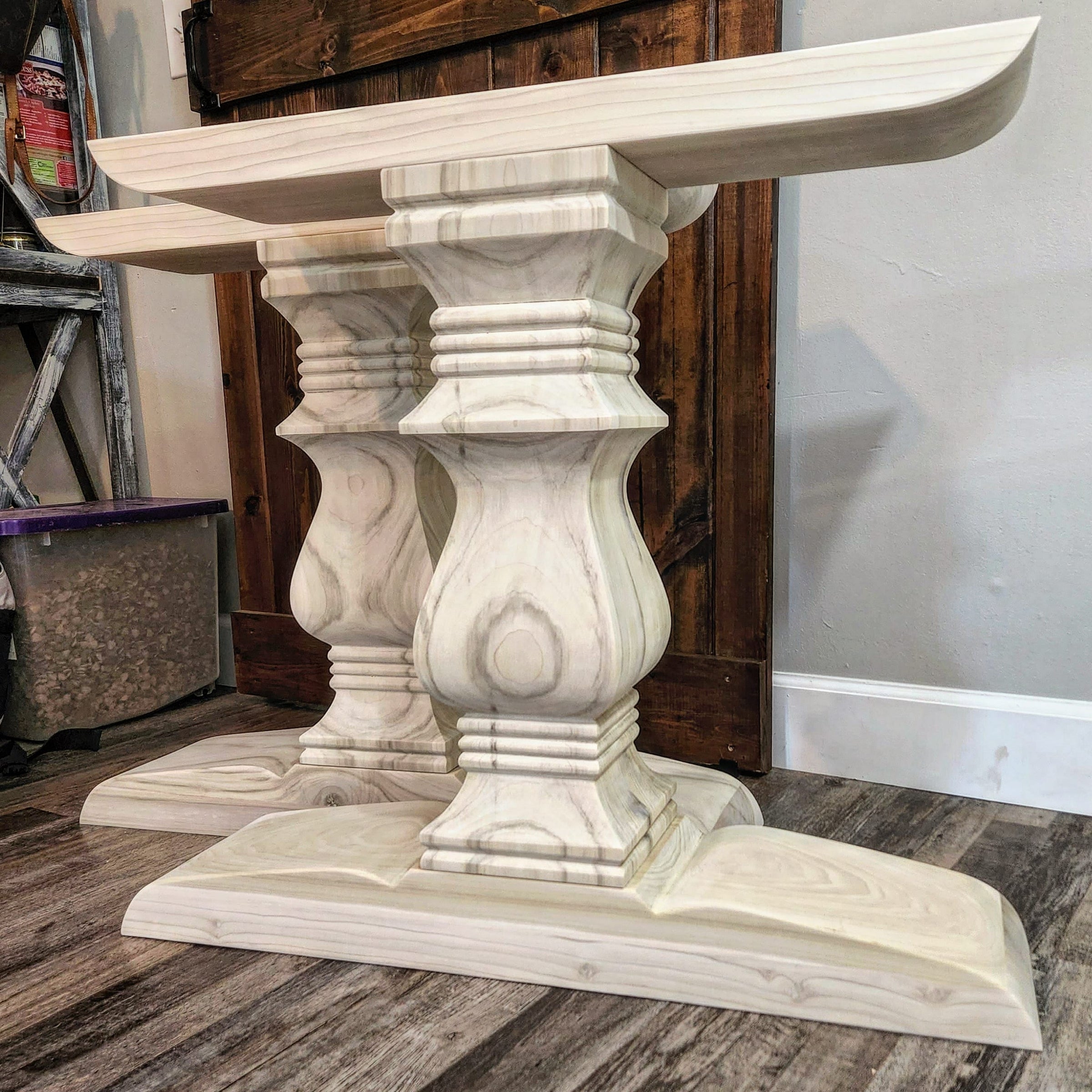This image showcases two paired, unfinished wooden table legs, featuring intricate craftsmanship and an antique style design. The legs, large and raw with an ashy, light brown color, exhibit a detailed curvature reminiscent of an hourglass half. These curves are bookended by rectangular segments at the top and bottom, giving them a sophisticated, corbel-like appearance. Each leg has a flat piece at both the top and bottom, hinting at their potential as sturdy supports for a table or desk. The legs rest on a grayish-brown wooden floor, echoing the rustic theme. In the background, there is a dark brown wooden door or tabletop. Additional contextual elements include a clear container with a purple lid filled with dog kibble and a possible metal shelf structure on the left, which adds to the busy, workshop-like setting. The wood's natural knots and grain give the legs a marble-like appearance, enhancing their aesthetic appeal.